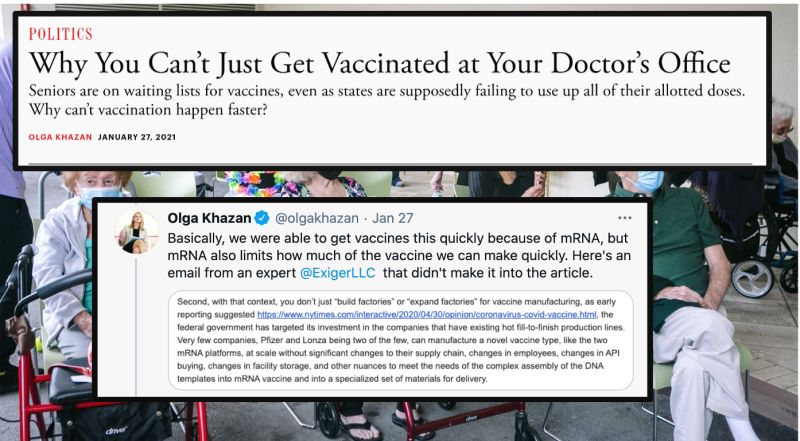This image is a detailed screenshot from an unspecified website, as neither the header nor the footer are visible. The background features a photograph of elderly individuals using walkers and wheelchairs. On the left, an older white woman with reddish-brown hair, seated on a walker with a seat, is wearing a surgical mask. On the right, only the bottom half of a man's face is visible; he is also wearing a surgical mask, is dressed in a green shirt and white pants, and has his legs crossed.

Superimposed on this background are two rectangular text boxes. The larger, top rectangle, outlined in black and red, is centered at the top. Inside it, the left side is labeled "POLITICS." The headline reads, in large black font: "Why You Can't Just Get Vaccinated at Your Doctor's Office." Below the headline, in smaller font, the subtext states: "Seniors are on waiting lists for vaccines even as states are supposedly failing to use up all of their allotted doses. Why can't vaccination happen faster?" The author’s name, Olga Khazan, appears in red capital letters. The article is dated January 27, 2021, written in black capital letters.

Below this is a second, smaller white rectangle containing a Twitter screenshot. The tweet is from the same author, @O_Khazan, recognizable by her profile photo where she has blonde hair and is wearing a light-colored top, potentially a sweater, paired with a black mini skirt or dress. The tweet, dated January 27, explains, "We were able to get vaccines as quickly because of MRNA but MRNA also limits how much of the vaccine we can make quickly. Here's an email from an expert." Following this, the tweet references an email from an expert at EXIGER LLC, and includes a lengthy quote from the source, mentioning a hyperlink to a New York Times article.